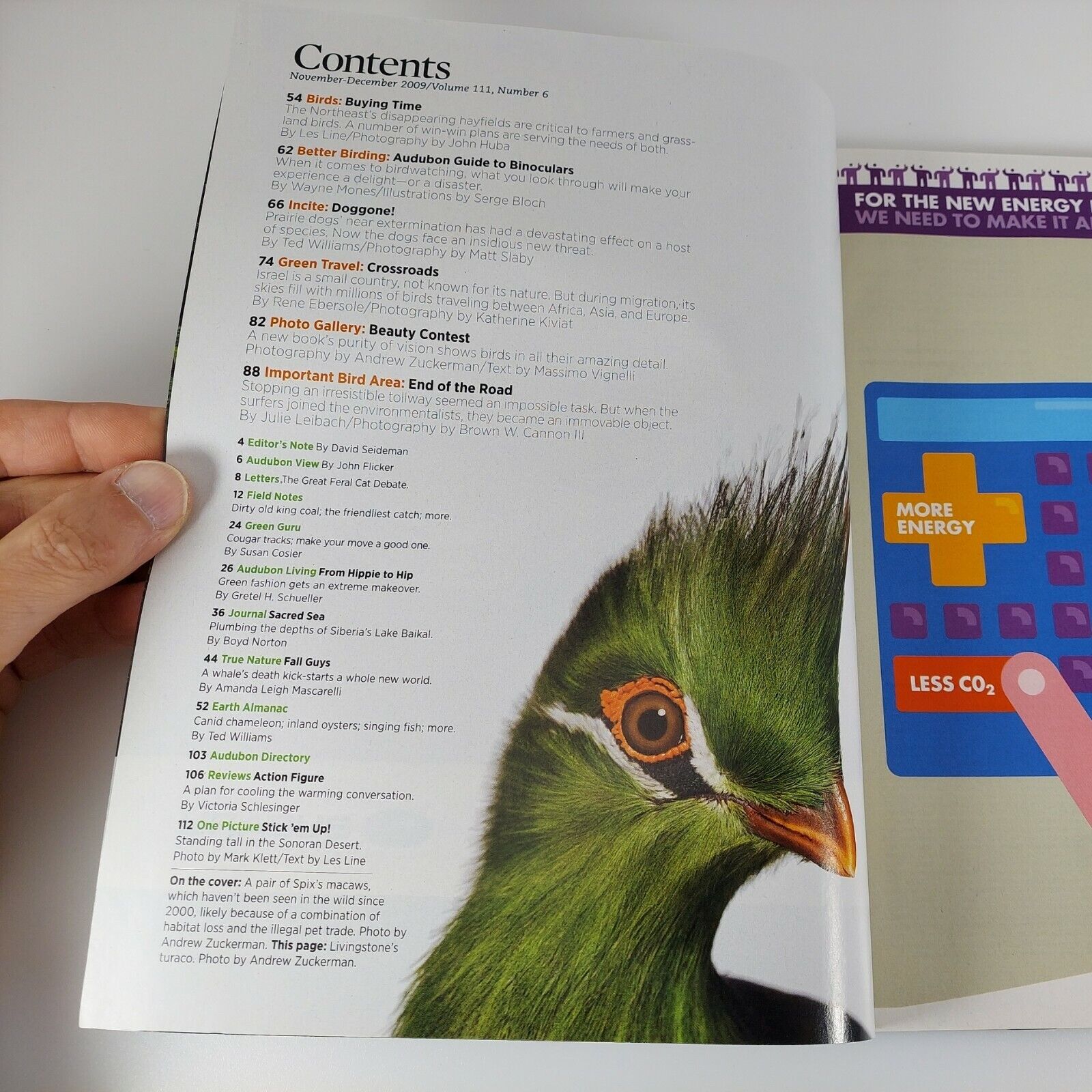In this detailed photograph, we see a man's hand entering from the left side, holding open a folded magazine to the contents page, set against a clean white background. The magazine is from November to December 2009, Volume 111, Number 6. Prominent on the contents page is a vibrant image of a large green bird, featuring an orange beak, brown eyes with orange fur around them, and black and white stripes. This bird is situated in the bottom-right section of the page. The content headings are styled in black text with some orange highlights, and green accents are also present at the bottom. The magazine features sections such as "Birds," "Better Birding Insight," "Green Travel," "Photo Gallery," "Important Bird Area," "Editors Notes," "Letters," "Field Notes," and "Green Room." To the right of the magazine sits a book accompanied by a top-flipping spiral notebook. Through the open page, one can discern an advertisement on the following page, promoting "more energy and less CO2." The clean layout and detailed focus on the bird and contents highlight the magazine's dedication to ornithology and environmental themes.